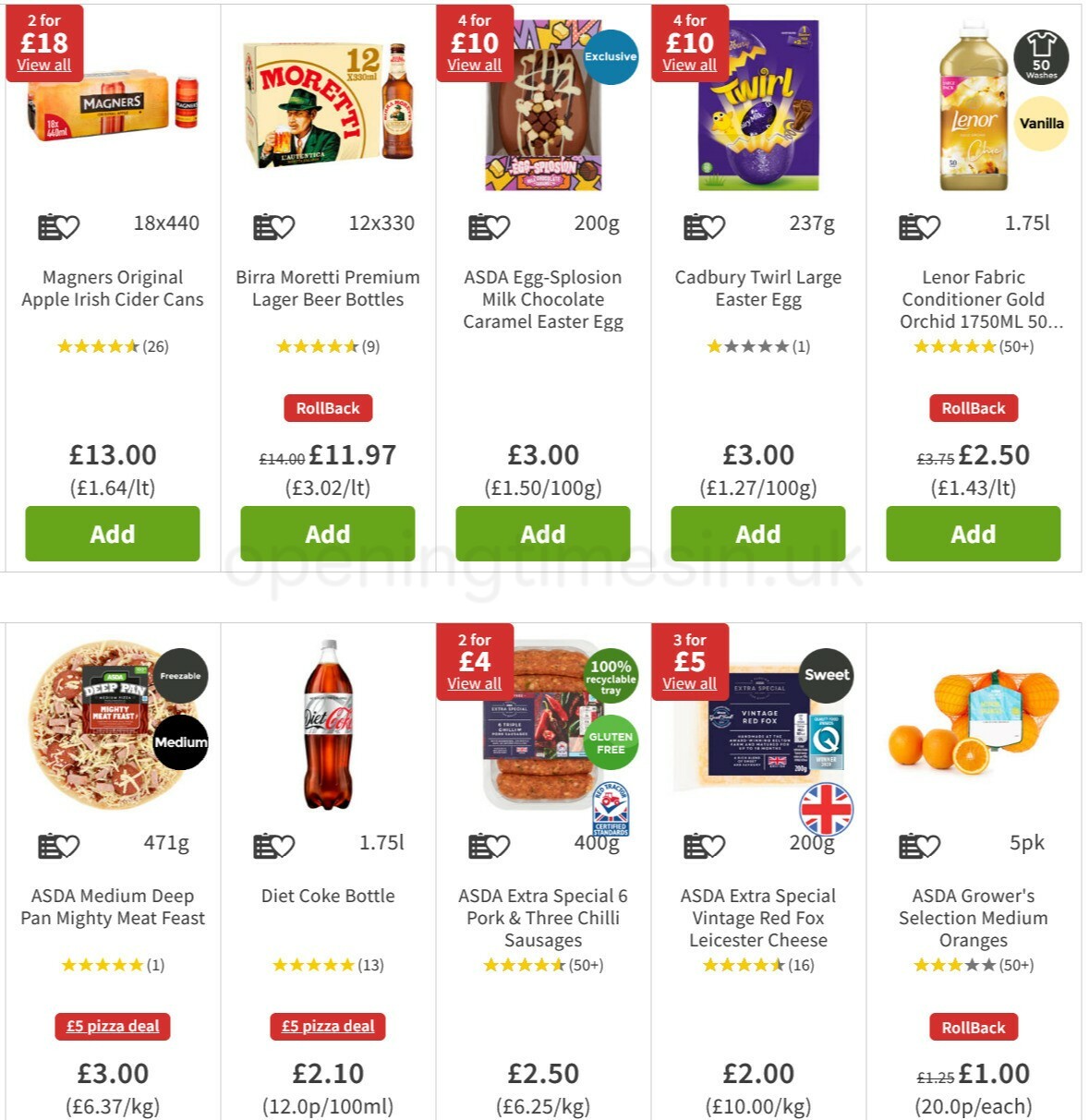The image depicts a screenshot from an online grocery store interface. The background is predominantly white and is segmented into two rows, each displaying a selection of products in long, narrow, vertical rectangles. Each product listing includes a product image, description, price, and an “Add” button, which is green.

In the top row, the first product on the left is Magners Original Apple Irish Cider Cans. The listing features a yellow box with the Magners logo and a can of cider beside it. The price is listed as £13.00, and a green "Add" button is located at the bottom of the rectangle.

To the immediate right of the cider, the next product is Birra Moretti Premium Lager Beer Bottles. The image shows a carton labeled with the number 12 and the Moretti logo, which includes a depiction of a man with a green hat drinking beer. A bottle of the lager is pictured next to the carton. The price is £11.97, and this listing also includes the green "Add" button at the bottom.

In the bottom row, the second product from the left is a Diet Coke bottle. The description reads “Diet Coke Bottle,” and the price is £2.10. However, the green "Add" button at the bottom is partially cut off in all products shown in this row, making it not fully visible.

Overall, ten products are displayed in the image, but only the specific details of Magners cider, Birra Moretti beer, and Diet Coke are clearly described.